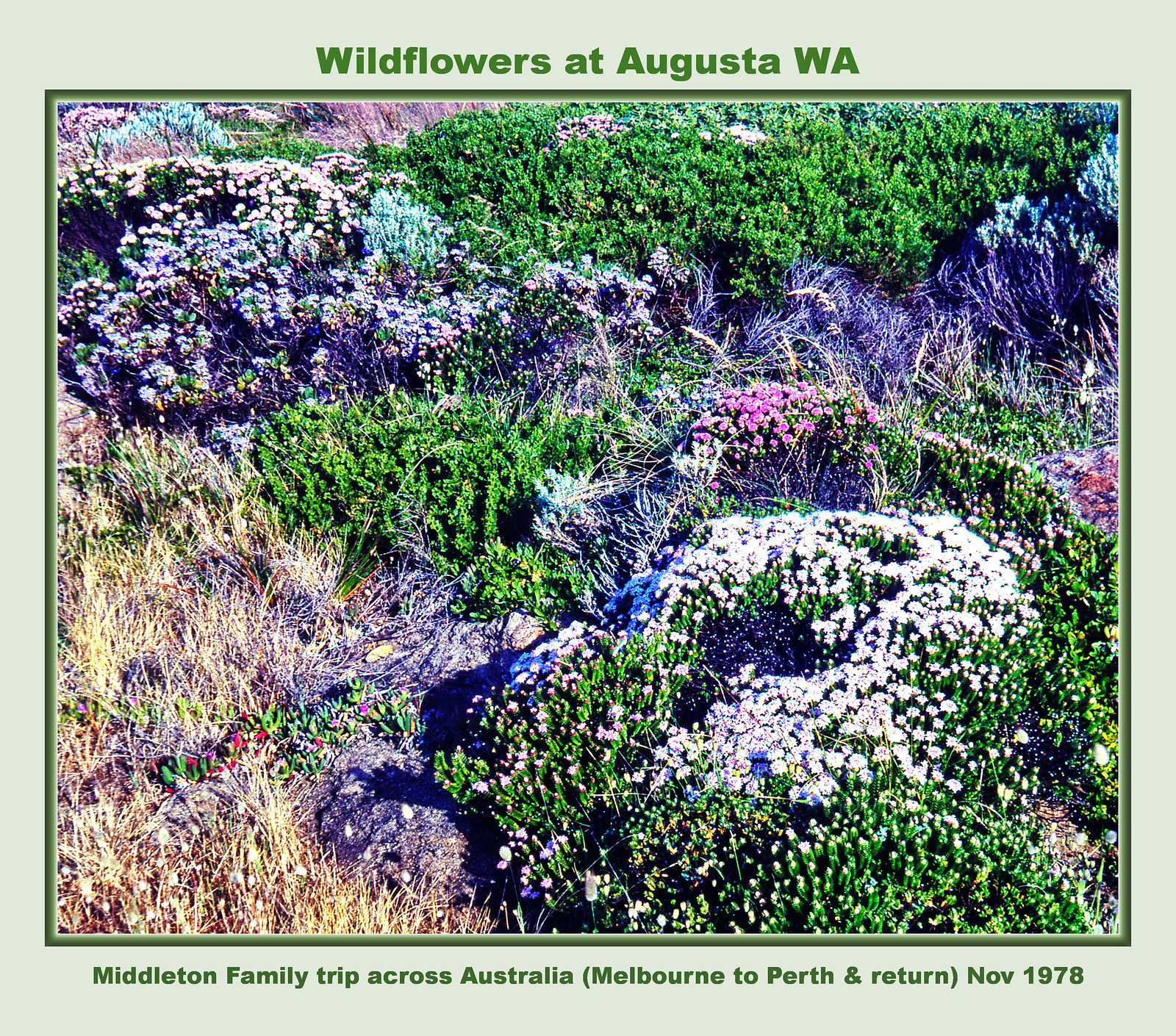This vivid photograph, titled "Wildflowers at Augusta, Washington," and captioned "Middleton Family Trip Across Australia, Melbourne to Perth and Return, November 1978," captures an abundant field of diverse vegetation. In the foreground, numerous bushes, some adorned with white, pink, purple, and blue flowers, are interspersed with vibrant green foliage. Brown grass stretches throughout the scene, where low-lying vines bear red berries, adding texture and color contrast. The overall setting appears lush and full, suggesting it’s spring or summer. The image, although chaotic with elements like dead branches, evokes a serene and natural ambiance. Enhanced details bring out the colors vividly, making the scene feel almost surreal.